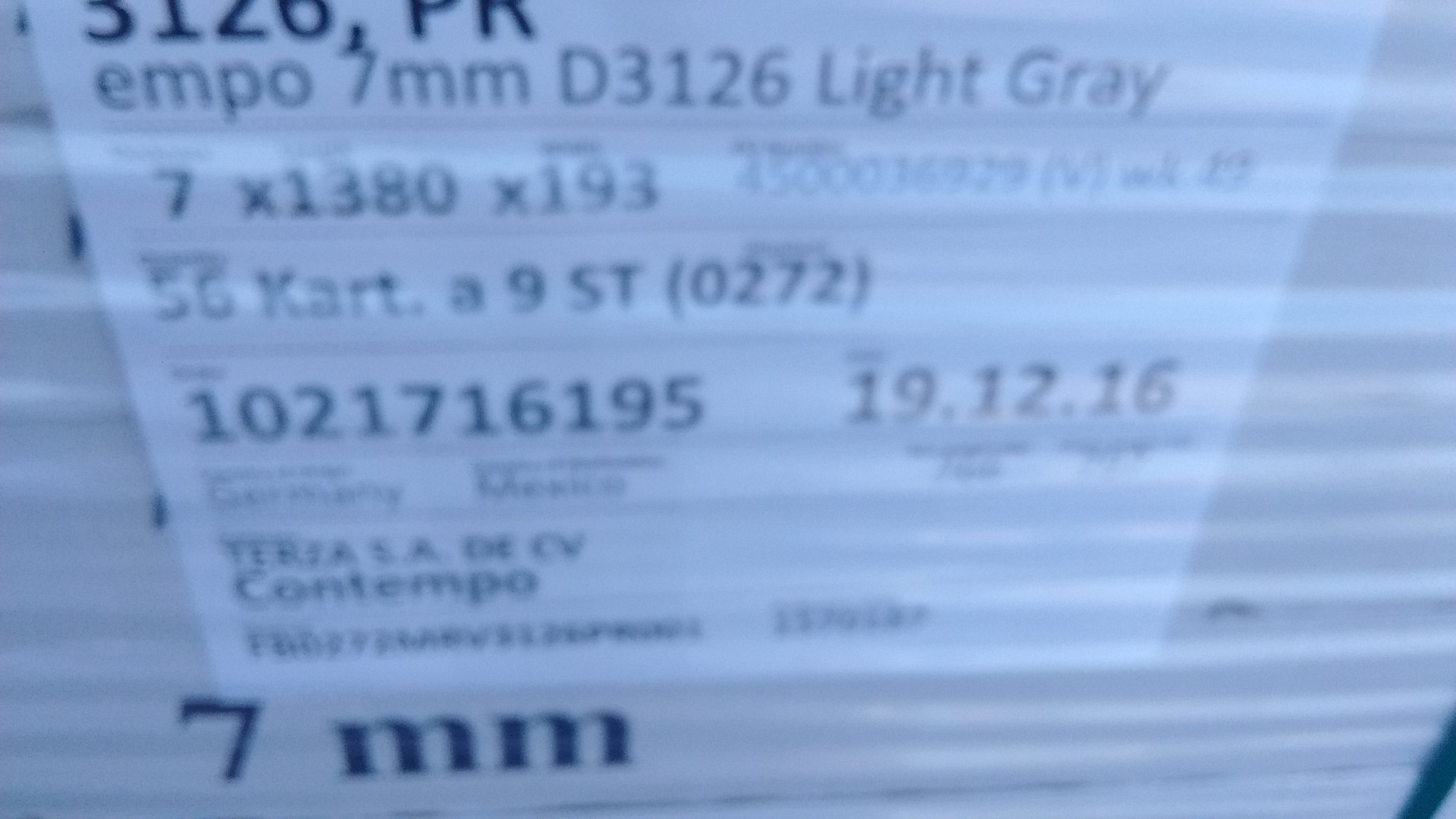This detailed caption describes an image of a packing label with various data points and information. 

---

The image showcases a packing label with an alternating light grey and dark grey striped background. At the top of the label, there is some dark print that is partially obscured, rendering only half of the text visible. Beneath this segment, a product code "EMPO 7MMD3126" is clearly printed in light grey.

Below the product code, dimensions "7 x 1380 x 193" are listed, indicating the size of the enclosed product. Adjacent to these dimensions, partially faded numbers read "45000," though the remainder of these figures is too faint to decipher.

Further down, the label reads "56KART.A9ST 0272," followed by another string of characters including "1021716195 19.12.16," which likely represents a date. Continuing lower, there are more letters, and prominently features the word "CONTEMPO."

Centrally placed in bold, large type is the character set "7MM," standing out prominently among the other textual elements.